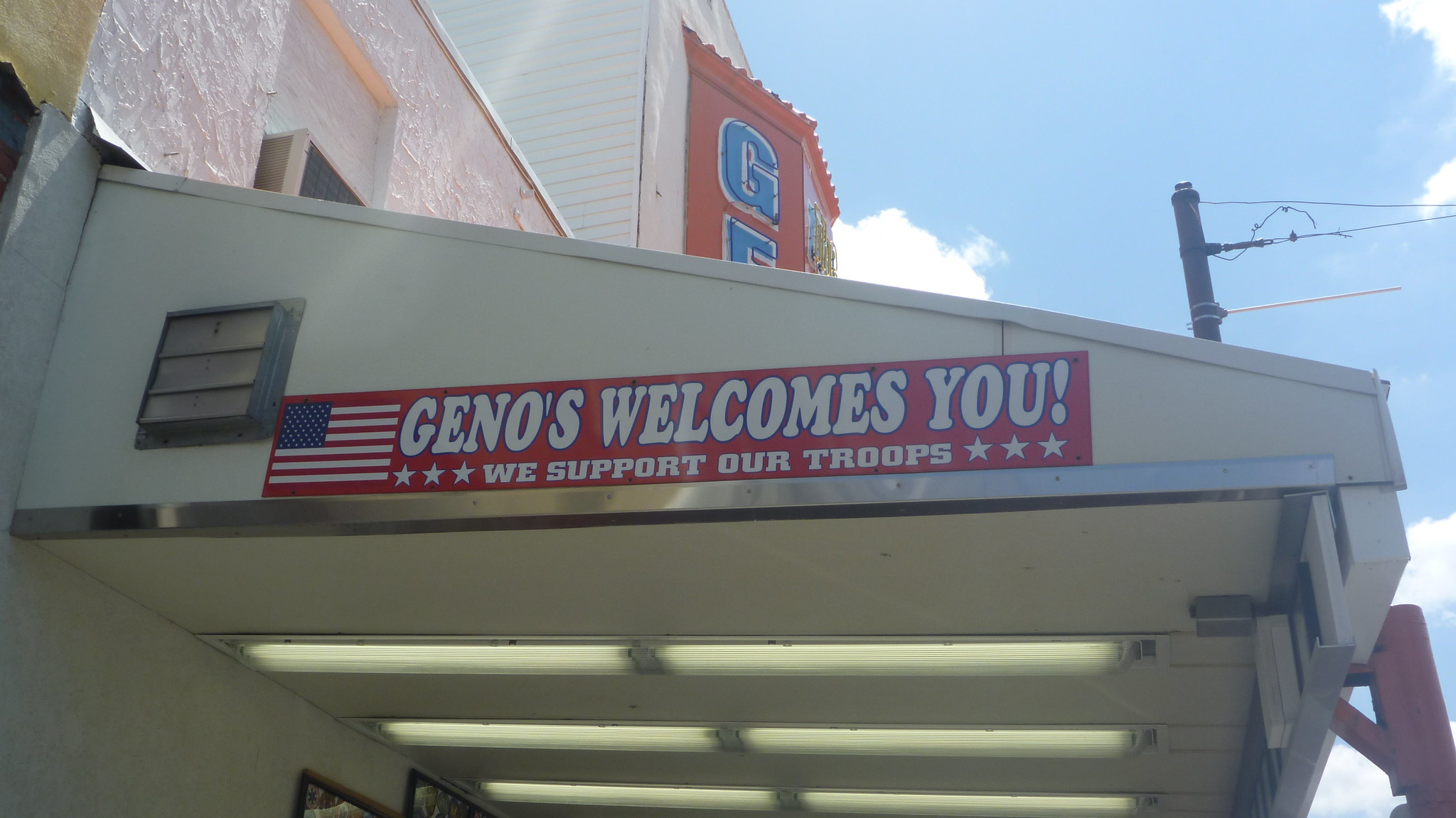The photograph captures the white awning of a store, possibly a restaurant named Gino's, taken from a side angle during the daytime. Mounted on the side of the awning is a horizontal, dark red sign bordered in a rectangle shape, which prominently displays "Gino's welcomes you" in big white text flanked by three white stars on each side. Below, it reads "We support our troops," with an American flag situated on the left of the sign, highlighting the patriotic theme. Above the awning, partially visible against a reddish-orange backdrop, are the blue neon letters "G" and "E," suggesting a larger sign spelling "Gino's." Numerous vertical lights adorn the roof part of the awning. In the background, there’s a glimpse of a piece of blue sky in the top right corner, and an electricity post with power lines is also visible on the right side of the image.